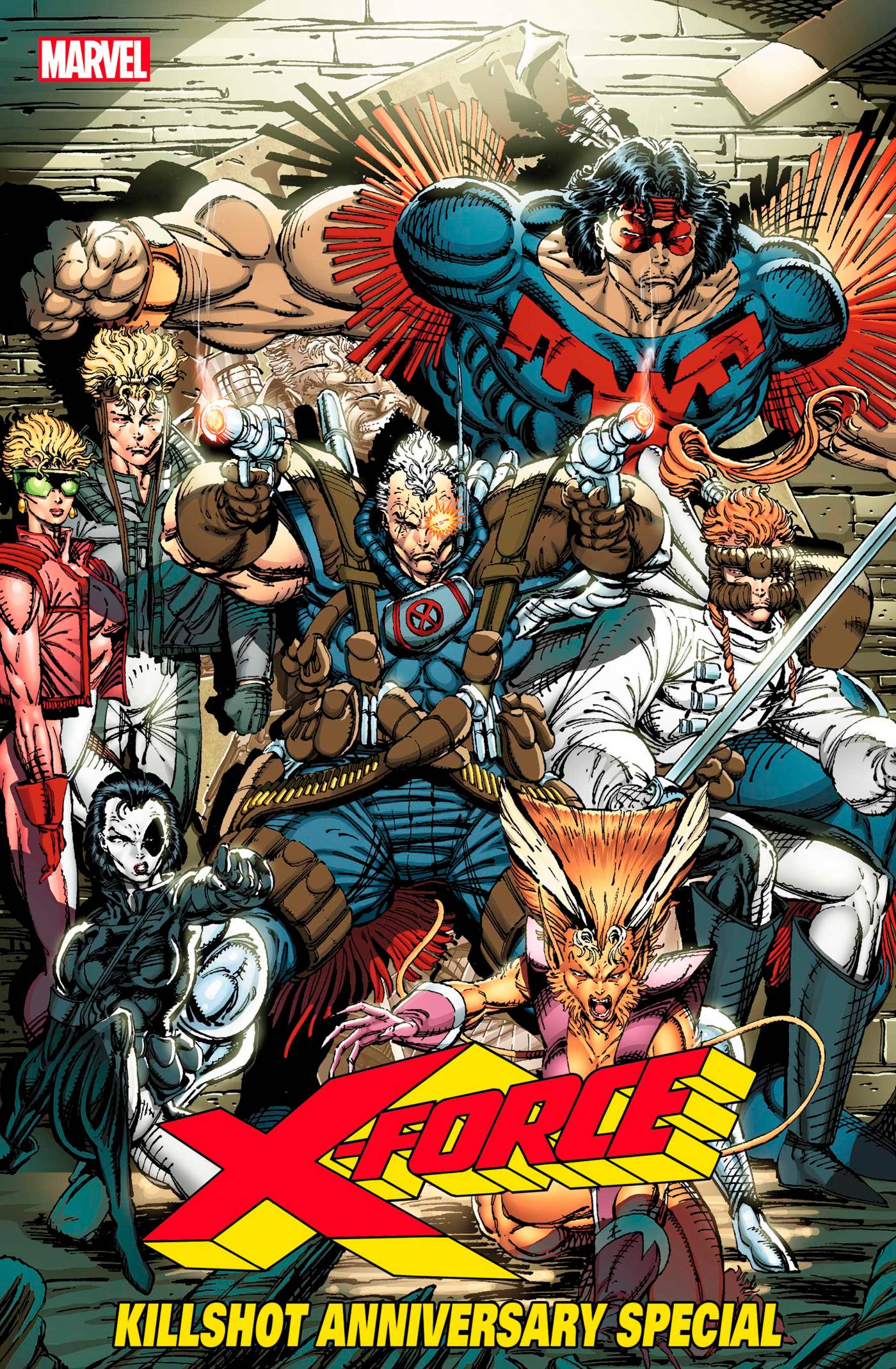The cover of this Marvel comic book titled "X-Force Killshot Anniversary Special" is striking and loaded with detail. The "Marvel" logo is placed in the top left corner within a red box. Dominating the scene is a massive, muscular character bursting through a backdrop of grey stone wall. This character wears a blue skin-tight suit with red fringes around his short sleeves, long black hair, and a red face mask. Below this formidable figure, other characters are depicted, creating a busy and dynamic composition.

In the center, a slightly smaller muscular man in a blue skin-tight suit, accentuated with brown straps, holds silver guns. This character also features an orange glowing eye, adding a dramatic touch. Positioned to his right is a person clad in a white outfit with a brown face mask, sitting in a chair. To the left of the central figure stands a woman in a pink vest, sporting trapezoid-shaped, cat-like orange and white hair.

In the bottom left of the cover is a woman with a white face and a black oval over her left eye, slicked-back black hair, and a skin-tight black and white suit. Adjacent to her on the right, another woman is seen wearing a pink vest with similar orange and white hair. 

At the bottom of the cover, in bold red text with a yellow outline, the title "X-Force" is displayed prominently. Beneath it, the subtitle "Killshot Anniversary Special" is presented in yellow text. The entire scene is populated with characters displaying aggressive and determined expressions, all incredibly muscular and positioned strikingly against the grey stone wall.